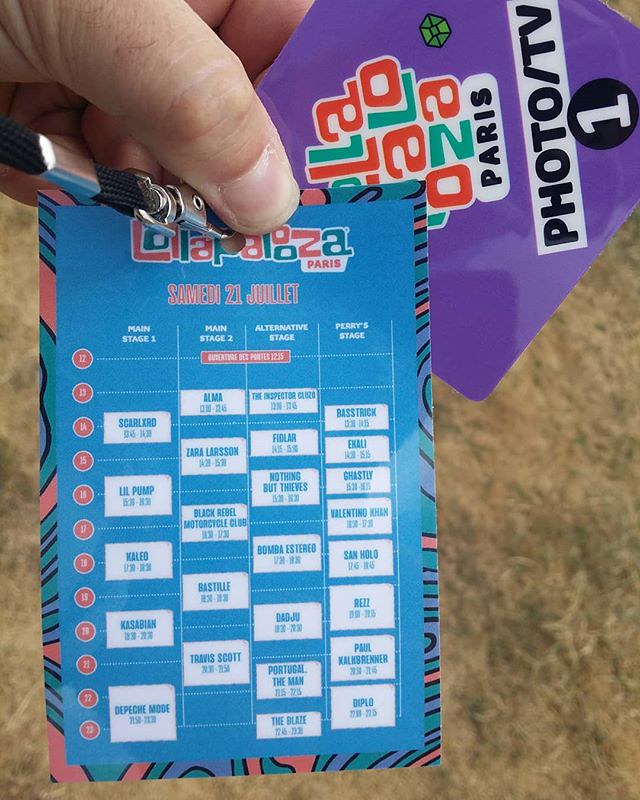The image is a detailed photograph showing a lanyard holding two cards, prominently featuring a blue card in the foreground. A person's thumb and fingers are visible gripping the blue card at the top left. The blue card has a thin border with black and red lines, displaying "Lollapalooza" in red and blue letters at the top, followed by "Paris." Below this, in smaller red print, it reads "Samadhi 21 Juillet." The card is sectioned into four vertical columns labeled "Main Stage 1," "Main Stage 2," "Alternative Stage," and "Paris Stage," each with rows of information. Red numbers in circles ranging from 12 to 23 are aligned vertically along the left side, with corresponding rows of white boxes filled with blue text.

Behind the blue card, a purple card can be seen partially, oriented sideways. It reads "Lollapalooza" in three lines with "Paris," and "photo/TV" underneath, ending with the number "1" in a black dot. The background of the image is out of focus, appearing as a textured mix of brown, black, and white, resembling carpet. The photograph captures the detailed arrangement and text on the cards, suggesting they are passes or schedules for an event, likely the Lollapalooza festival in Paris.